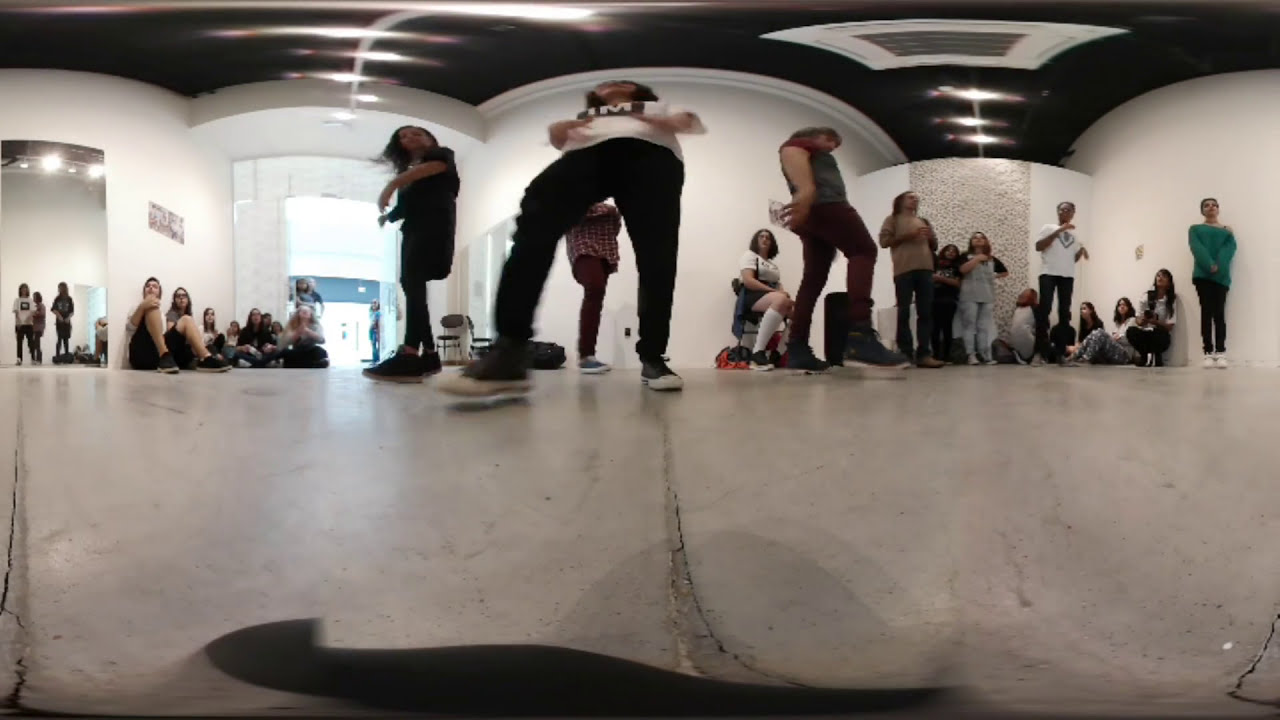This captivating photo captures an indoor scene, likely within a dance studio, featuring a group of people who appear distorted due to a warped camera effect, possibly from a 360-degree lens. The room has striking white walls and a black ceiling, adding to the stark contrast in the environment. The concrete floor supports a dynamic scene in the center where four people—all dressed in varied clothing from dresses to pants and flat shoes of different styles—engage in dance-like movements. The person in the center stands out with black pants and a white shirt, flanked by a person in all black on the left and another in a green shirt with burgundy pants on the right. Surrounding them, other participants are seated or standing against the walls, also twisted by the optical distortion, observing the central figures. A mirror on the left reflects the scene, enhancing the sense of space. The far background reveals a brightness coming from what seems to be glass doors leading outside, indicating daylight. The varied colors and the room’s layout suggest a lively and spontaneous moment captured amidst a lesson or performance, compelling the viewer to engage with the unusual, surreal aesthetic created by the warped imagery.